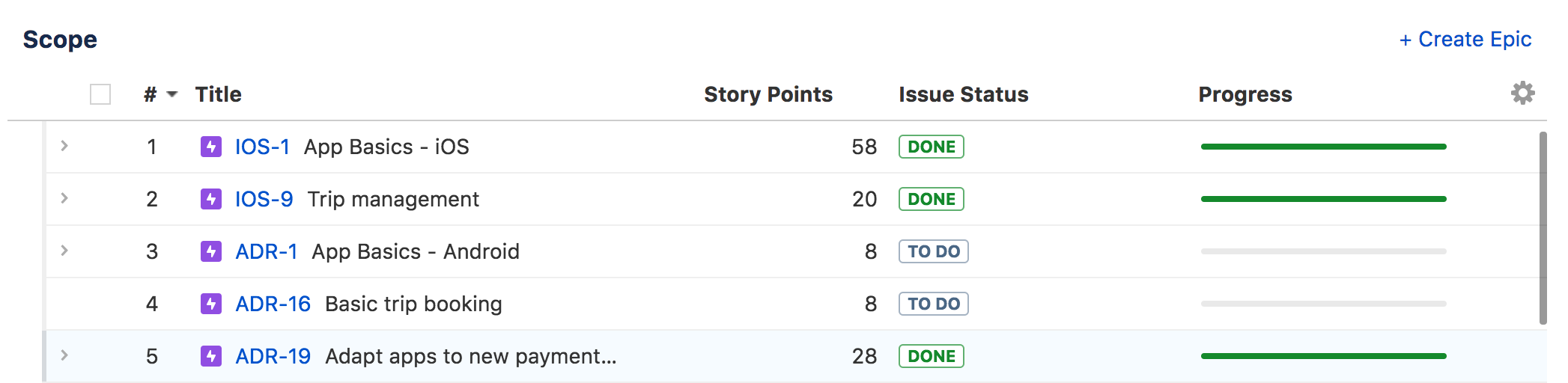The image features a detailed outline of a structured training or project management program. The top left corner is labeled "Scope," suggesting an overview of objectives or tasks to be accomplished. The scope is divided into five key items, presented in a table format:

1. **iOS: Basics** - This item comes first in the sequence. It appears to be a fundamental course or module focusing on basic iOS functionalities. It is marked with 58 story points and is noted as "Done," with progress marked as "Completed."
  
2. **Trip Management** - The second item on the list. While exact details are not provided, it likely involves learning or managing trip-related tasks.

3. **Android: Basics** - The third item, similar to the first, but focused on the Android operating system. Its progress is still pending, highlighting that this part of the curriculum or project is yet to be completed.

4. **Basic Trip Booking** - The fourth item, which seems to cover the basics of booking trips. This also remains incomplete, listed with 8 story points.

5. **Adopt Apps to Do Payment** - The fifth item, focusing on integrating or utilizing apps for payment processing. The progress status of this item is not explicitly mentioned.

Each task or module is associated with reference numbers, story points (indicating the effort or complexity involved), and issue statuses (tracking progress). This setup seems oriented towards IT training, customer support training, or a project management scenario where individuals must complete these foundational tasks before progressing to more advanced responsibilities.